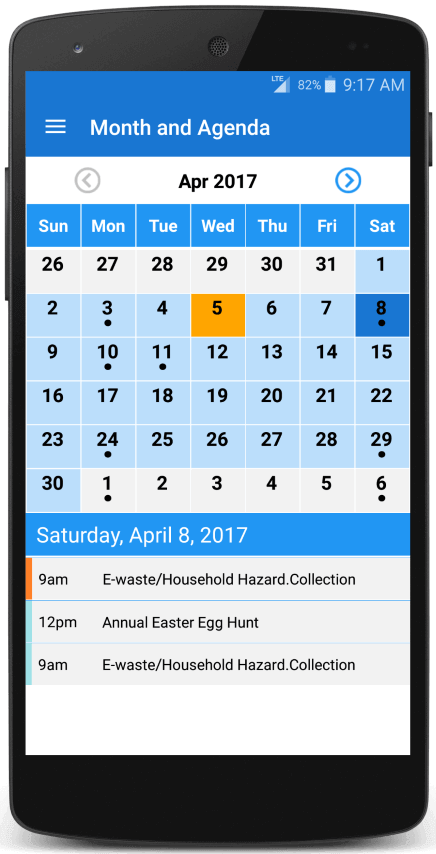A photo captures a sleek, portrait-oriented cellular device or PDA positioned against a white background. The device is rectangular with rounded top and bottom edges, and features a single button on the top right side and a large volume control button extending downward on the left. A blue horizontal border spans the top of the screen, displaying a white hamburger menu icon, and the text "Month" and "Agenda" in white font. The network connection shows LTE above the signal bars, with a battery life indicator at 82%, and the time displayed as 9:17 AM.

Beneath this, a white horizontal bar allows for scrolling through months, currently set to April 2017 in black text. Arrows for navigating between months are present, with the back arrow grayed out and the forward arrow in blue. Below this, a calendar layout presents the days of the month in column format. Days of the current month are highlighted in blue with dots indicating events. Previous months' days, falling within the calendar view, are in gray with black text.

Specific attention is drawn to Wednesday, April 5th and Saturday, April 8th, which are color-coded—orange for April 5th and blue for April 8th. The schedule for Saturday, April 8th is displayed below, detailing two events: "9 a.m. e-waste household hazard collection" and "12 p.m. annual Easter egg hunt." Additionally, "9 a.m. e-waste household hazard collection" is repeated, indicating the event's significance or recurrence.